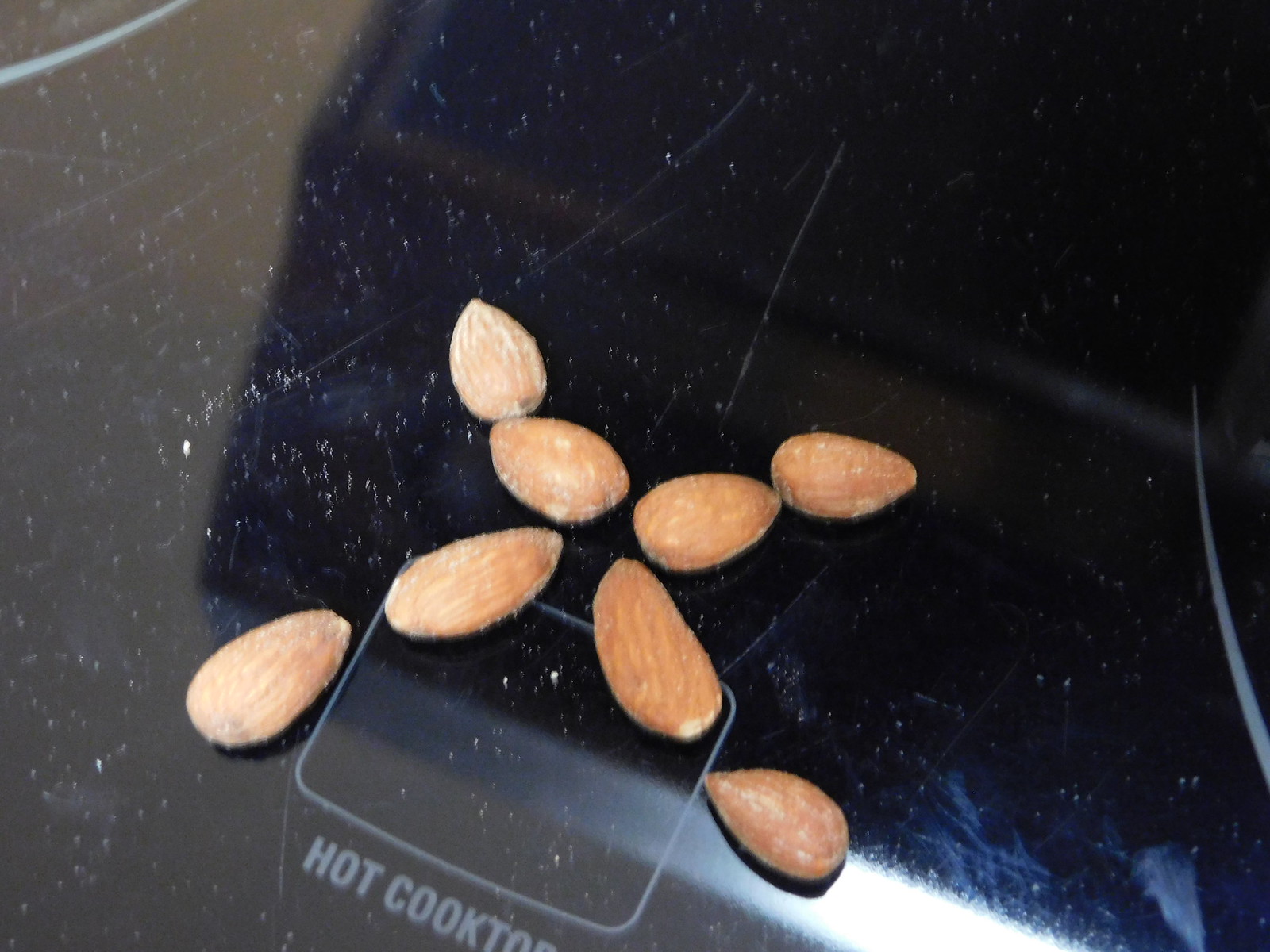In this color photograph, eight brown almonds are arranged in an X shape on a black stove surface. The stove is noticeably dusty and covered with a fine grainy material, likely salt, along with visible scratches and fingerprints, indicating it is not clean. The words "hot cooktop" are engraved in white just below the X of almonds. The rectangular design near the bottom left corner of the image, also in white, further identifies this as part of a stove's cooktop area. The stove surface's condition and the specific arrangement of the almonds contribute to a detailed and intriguing composition.